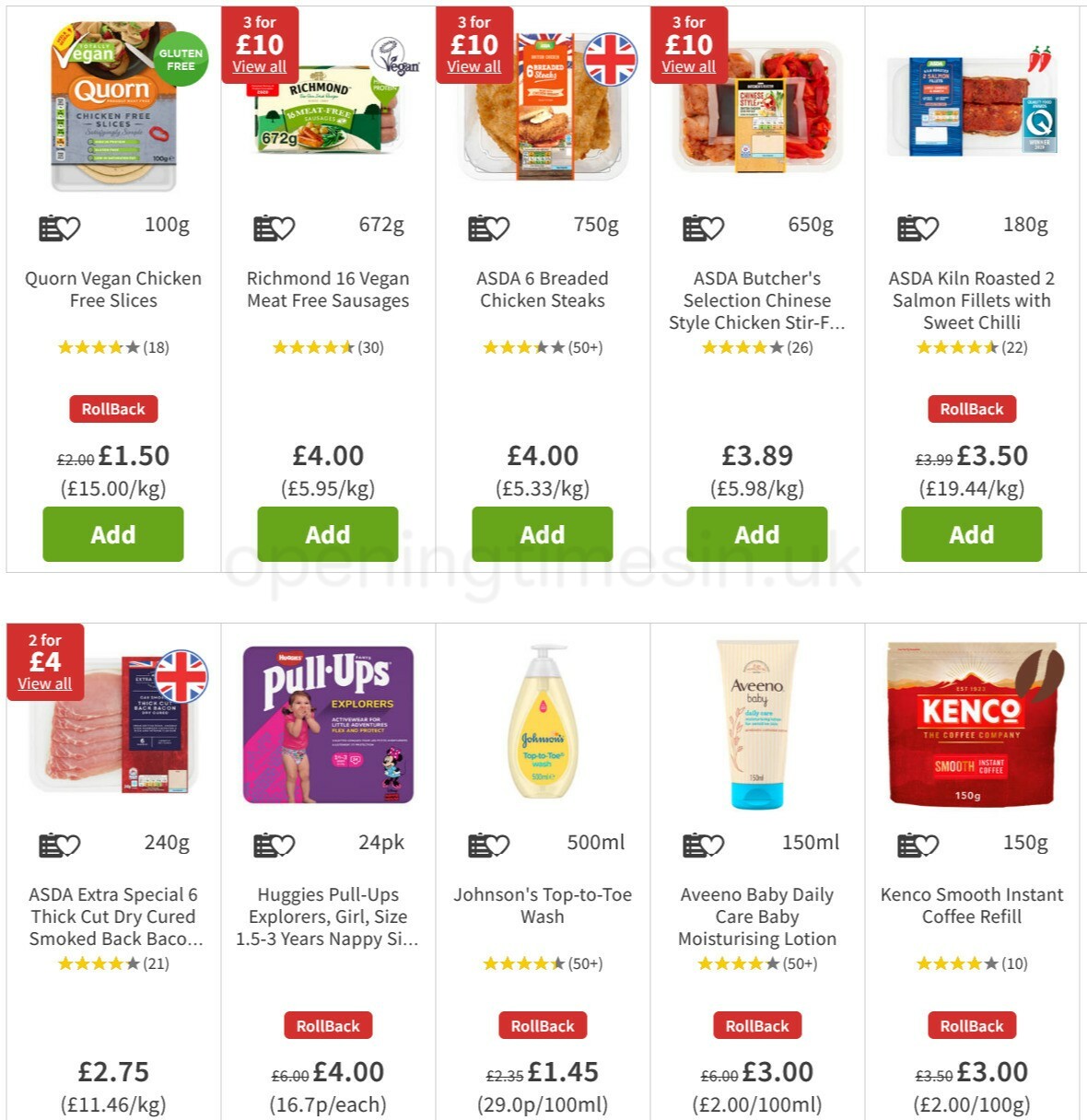This image depicts a page from a European online store where customers can order food and groceries. The layout features 10 rectangular boxes, each showcasing a different product with a clear, high-quality image. Among the items displayed are Johnson's Baby Shampoo, various salamis, bacon, and Aveeno Baby Moisturizing Lotion, which is notable for its upside-down blue cap. Additionally, there are Huggies Pull-Ups Explorers Girl Size diapers, suitable for ages 1.5 to 3 years. Each product listing includes prices in euros, with some items priced per kilogram, such as those listed at 15 euros per kilogram. The selection buttons for adding items to the cart are a distinct lime green color, enhancing the user interface for ease of use.